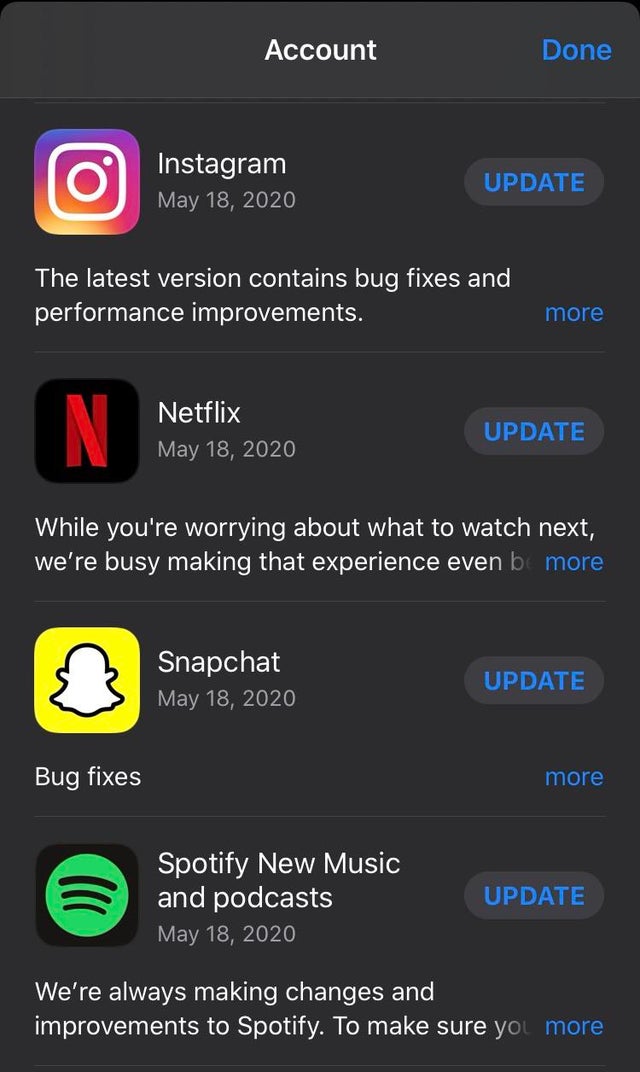A screenshot captured in dark mode from a mobile phone displays the account update page in an app store. The background is a dark grey, enhancing the readability of the white text. At the top, the category "Accounts" is prominently displayed. Beneath it, a section listing four apps—Instagram, Netflix, Snapchat, and Spotify—awaiting updates fills the screen.

Each app entry includes a "More" link for additional details and an "Update" button positioned on the right side. The specific update descriptions are as follows:
- **Instagram**: The latest version includes bug fixes and performance improvements.
- **Netflix**: "While you're worrying about what to watch next, we're busy making that experience even better."
- **Snapchat**: Bug fixes.
- **Spotify**: "We're always making changes and improvements to Spotify."

A "Done" button is located near the top right corner of the screen, indicating the user can exit the update view once they are finished. The vertical aspect ratio of the image confirms it was captured on a smartphone.